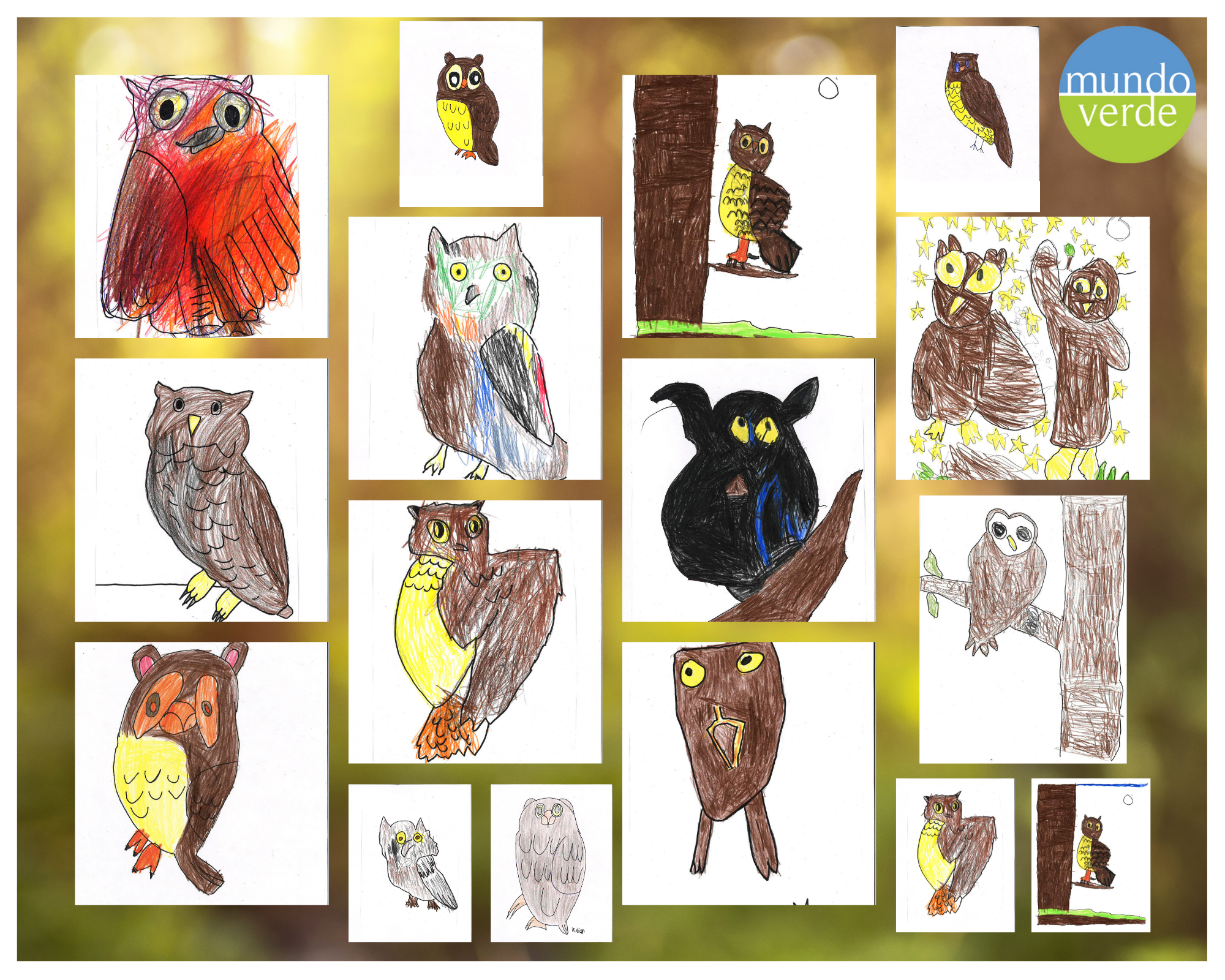The image showcases a charming collage of hand-drawn owl pictures, created by children using pencils and crayons. Against a brownish-yellow, slightly out-of-focus background, the collage features around 12 to 16 individual owl images, each on a white piece of paper. These drawings vary in size, color, and artistic style, showcasing a delightful mix of vibrant and understated hues, including shades of green, orange, red, yellow, blue, black, brown, and yellow. 

In the upper right corner, a circular emblem is divided into a blue upper half and a green lower half, with white text that reads "Mundo Verde." The drawings are arranged in four rows from top to bottom. Notable features include an orange owl with a black outline and large black eyes in the top left, a colorful owl with multiple shades such as green, orange, blue, red, and brown, and a variety of other owls in different poses and colors. Some owls are perched on tree limbs, and one image even features a person next to an owl with yellow stars in the background. The overall effect is a whimsical and heartwarming display of children's creativity and their interpretations of owls.